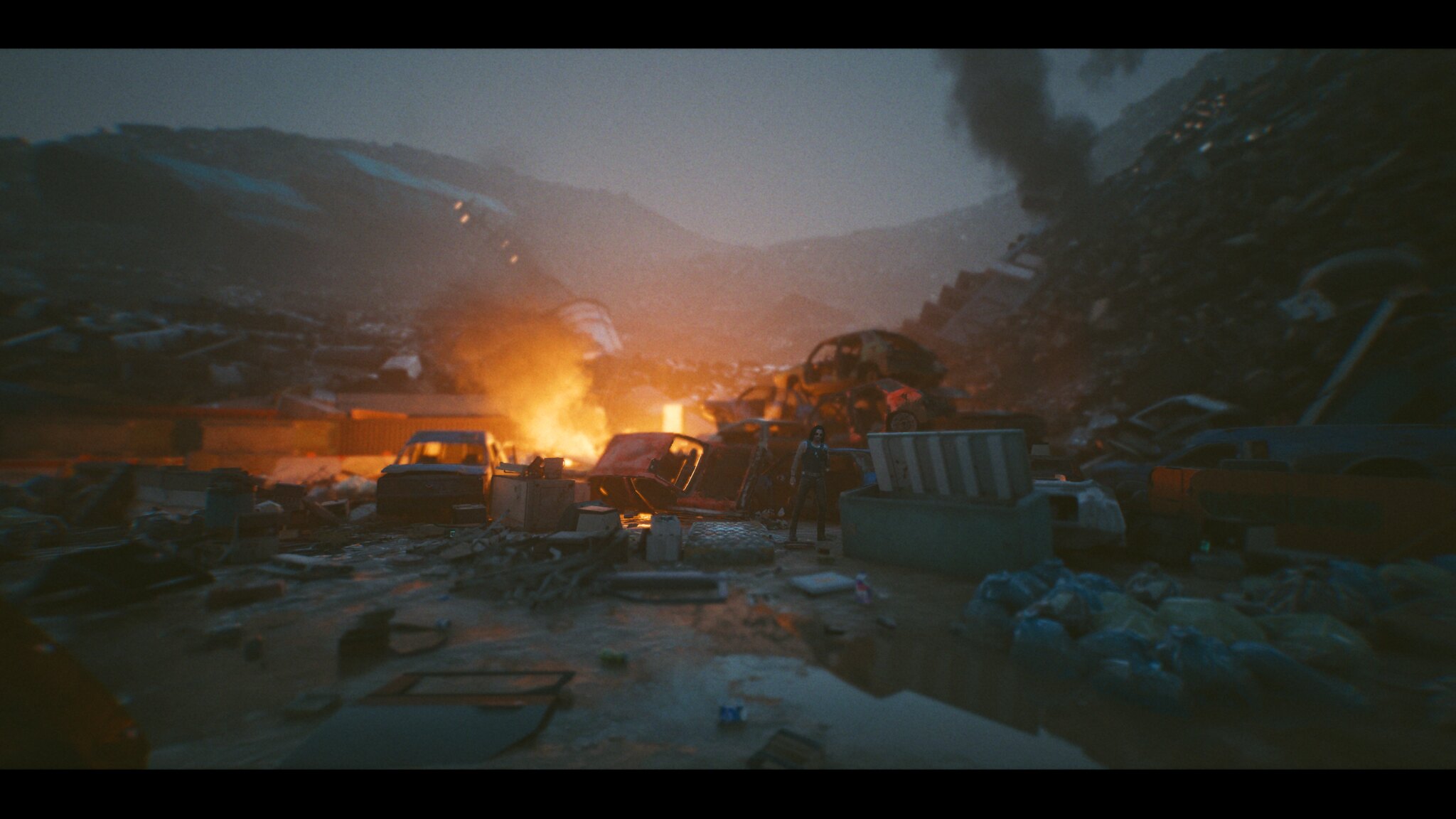The image is an incredibly realistic and dark screenshot, likely from a modern apocalyptic-themed computer game or possibly an AI-generated scene. The setting is a valley at night, flanked by towering, snow-dusted mountains that fade into a gray backdrop. The desolate landscape is littered with the remnants of civilization—burnt-out cars without windshields or tires, heaps of scrap metal, and an assortment of discarded human-made objects like sofas and boxes.

Towards the center of the image, a large, smoldering fire casts an orange glow, its white and gray smoke billowing upwards and dispersing into the air. This fire appears to be emerging from a pit-like area surrounded by more destroyed vehicles and rubble. Near the fire, slightly off-center to the right, stands a lone figure, possibly a woman with long hair, but the distance makes gender identification difficult. She wears a black outfit, perhaps a tank top, and dark blue jeans, staring directly towards the viewer.

The scene also features a dramatic crack in the earth near the right-hand side, with what appear to be blue and yellow bags—possibly garbage or body bags—strewn around it. The general atmosphere is one of complete devastation, emphasized by the pervasive gray tones, scattered debris, and omnipresent smoke. The image thoroughly encapsulates themes of destruction and human waste, contributing to a haunting and dystopian visual narrative.